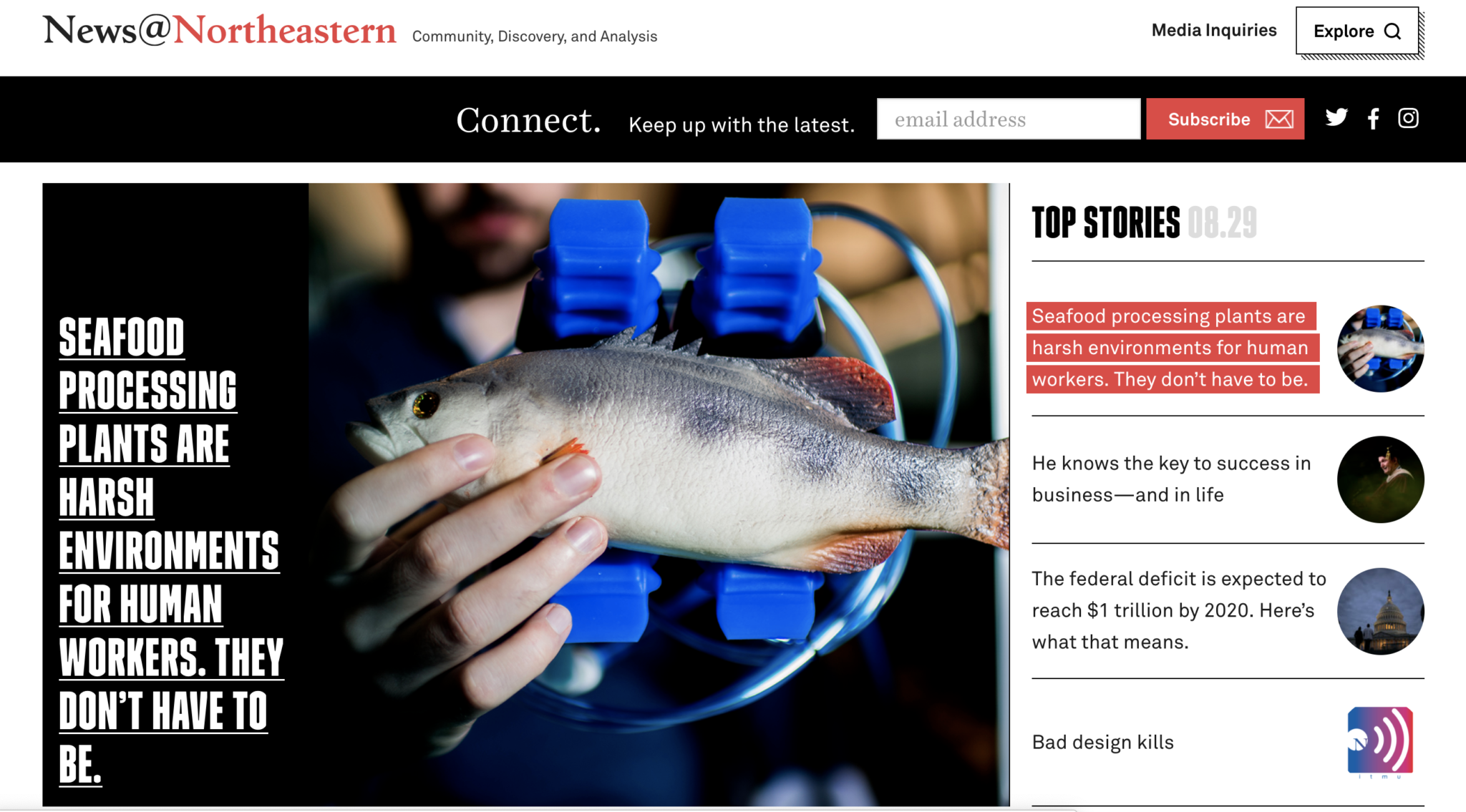In the upper left corner of the image, there are the headings "News at Northeastern," "Community," "Discovery," and "Analysis." Adjacent to these, there is a small rectangle that reads "Explore Inside" with a magnifying glass symbol inside. Below this, the word "Connect" appears with the phrase "keep up with the latest" and a field to input an email address for subscribing.

The main image depicts a man proudly holding a freshly caught fish out in a body of water. Behind him, various equipment including wires and a clamp are visible, suggesting a fishing or research-related activity. To the left of the image, a description highlights the tough conditions faced by workers in seafood processing plants, stating: "Seafood processing plants are harsh environments for human workers. They don't have to be." 

To the right, a series of story links and accompanying images are displayed:

1. The harsh environment of seafood processing plants is reiterated with the same statement.
2. Another story showcases a man within a circular frame with the caption: "He knows the key to success in business and in life."
3. A third story discusses the federal deficit, with the accompanying text: "The federal deficit is expected to reach $1 trillion by 2020. Here's what that means," illustrated with an image of a building inside a circle.
4. The final story has the stark warning "bad design kills," accompanied by an image that resembles a speaker or volume control inside a square.

This arrangement provides a visually engaging layout combining informative headlines with relevant images, offering a comprehensive overview of news and insights.